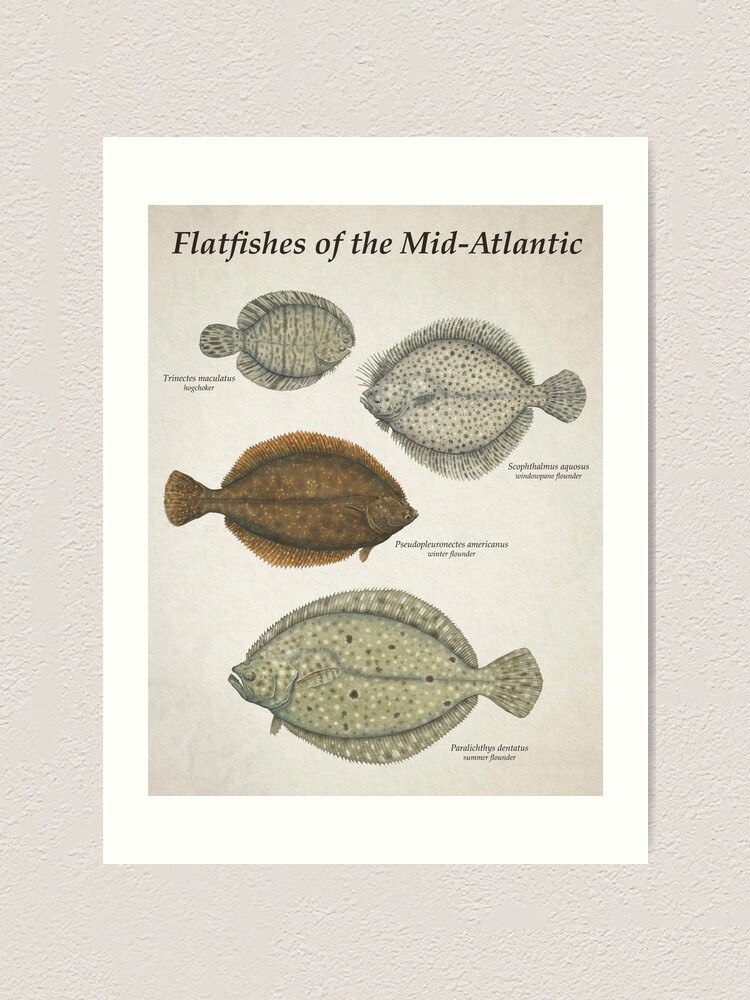A close-up photograph captures a detailed poster titled "Flat Fishes of the Mid-Atlantic," which appears to be slightly askew on a wall. The poster showcases various species of flatfish found in the Atlantic Ocean, each depicted with distinct illustrations. Due to the resolution, the names of the species are not legible. However, the visual details are clear:

1. The topmost fish is depicted in a light gray color, accented with dark blue lines.
2. Adjacent to it, the next species features a light gray hue with scattered dots.
3. Below, the third fish displays a dark brownish-orange shade adorned with light spots.
4. The bottommost and largest fish exhibits a dark greenish-gray color with distinctive spots.

Each species is meticulously illustrated, providing a comprehensive visual guide to the diverse flatfishes of the Mid-Atlantic despite the illegibility of their names.